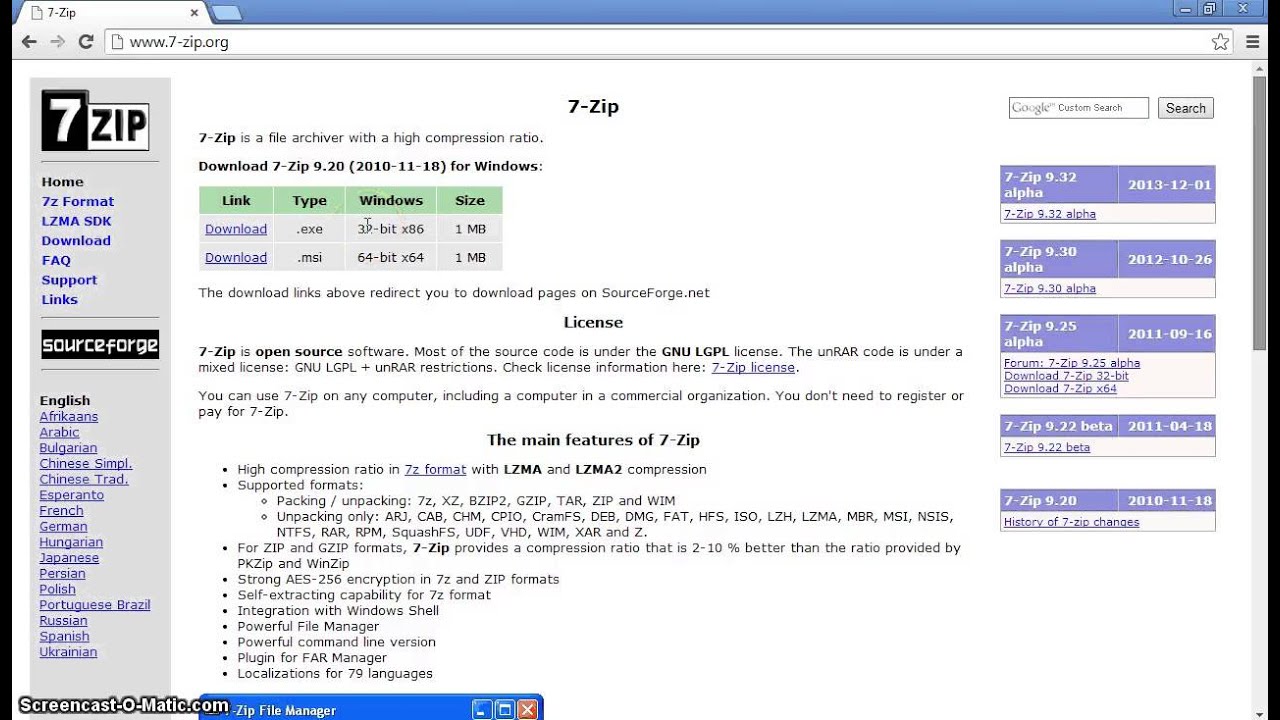The image features a white background with the website URL, "www.7-zip.org," prominently displayed. In the center, there's a bold "7-zip" logo placed above a gray rectangle housing a search bar. The text "7-zip is a file archiver with a high compression ratio" is clearly stated below. 

Towards the bottom, details for downloading 7-Zip version 9.20 (dated 2010-11-18) for Windows are provided. Below that, a table lists download link types. For "Type," it offers ".exe" and ".msi" file options. For "Windows," it specifies "32-bit x86" and "64-bit x64" versions, both with file sizes of 1MB each. Additionally, a cursor is shown hovering over the first download link, noting that these links redirect to source.net download pages. 

The image also emphasizes that "7-zip" is open-source software, with the majority of its source code available under the GNU LGPL license.